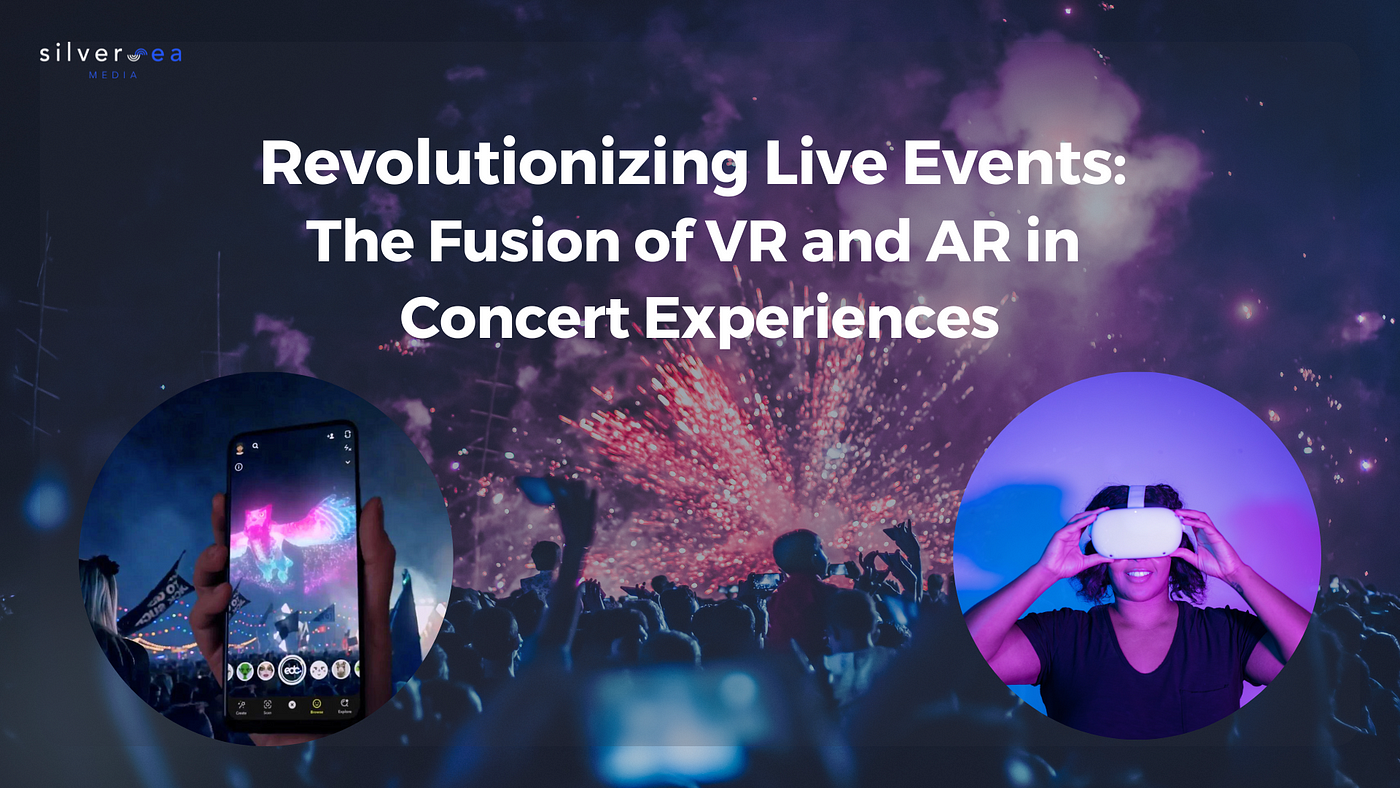This advertisement for Silver EA virtual reality glasses prominently features the company's logo in the top left corner, where “Silver” is displayed in white with a stylized blue "S" and "C," underlined by the word "Media" in blue. The centerpiece of the ad is a bold, white text proclamation: "Revolutionizing Live Events: The Fusion of VR and AR in Concert Experiences." The background showcases a vibrant scene from a music festival, depicting a sea of people amid fireworks and colorful lights, many capturing the moment with their phones. Overlaying this lively backdrop are two circular photographs. On the left, a person holds up their phone, seemingly using augmented reality features to enhance their concert experience. On the right, a woman with shoulder-length hair, wearing a black shirt, smiles as she enjoys the event using a sleek white VR headset. The juxtaposition of these images underscores the transformative potential of Silver EA's VR and AR technologies in live events.